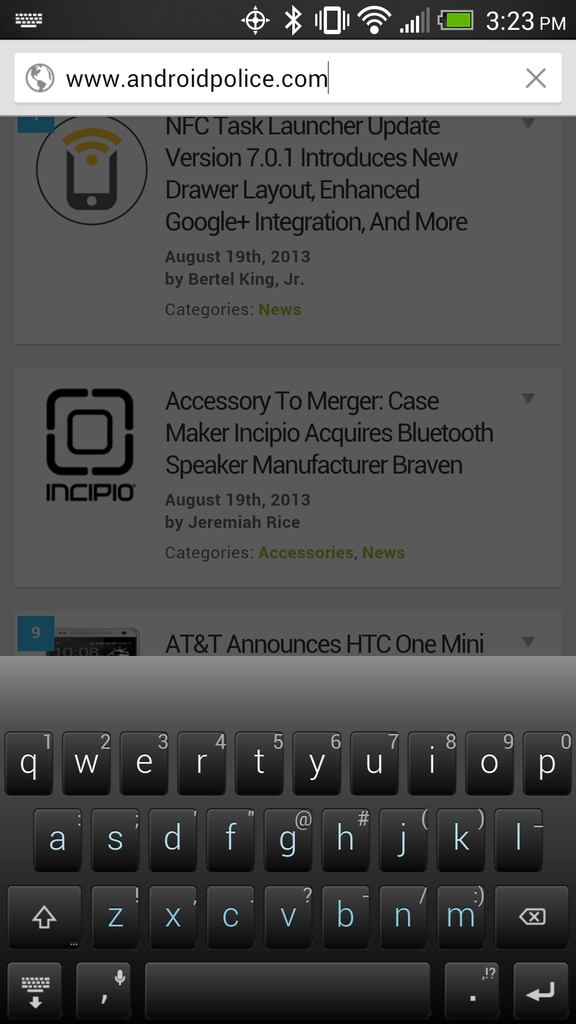A detailed caption for the described image:

"This screenshot appears to be taken from a smartphone and predominantly features a gray color scheme. At the very top, a black status bar is visible. To the upper left, there is a symbol that resembles a keyboard, which could be an indication of an active input method. On the right side of the status bar, the time is displayed as 23:00, accompanied by several other icons, including a green battery indicator and internet connectivity symbols.

Beneath the status bar, there is a white search bar. On the left side of this bar, an icon depicting a gray and white planet Earth is shown, followed by the URL 'www.androidpolice.com'. On the far right side of the search bar, there is a gray 'X' button.

Below the search bar, the screen transitions into a slightly darker gray area displaying text. The text includes headlines such as 'NFC task launcher update version 7.01 introduces new drawer layout, enhanced Google Plus integration, and more,' followed by another headline: 'Accessory to merger: Case maker Incipio acquires Bluetooth speaker manufacturer Braven.' The bottom portion of this area is cut off, truncating additional content.

At the very bottom of the screenshot, there is an on-screen keyboard. The keyboard layout is predominantly black, with the top row of keys displaying white letters and the middle and bottom rows showing letters in light blue. The space bar and additional function keys are also visible at the lower part of the keyboard."